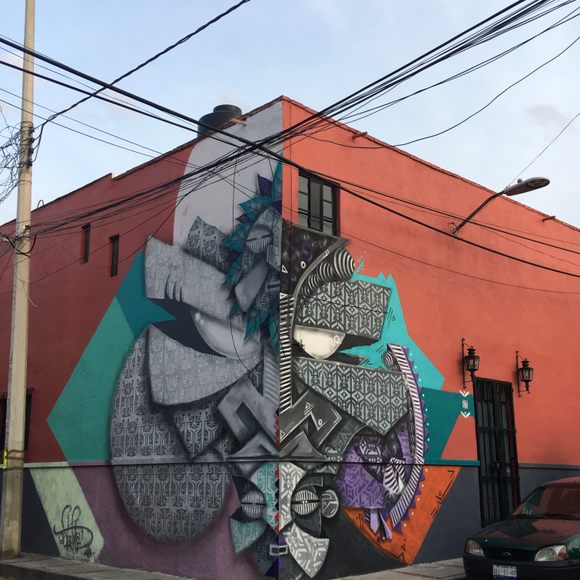The image features the corner of a maroonish-red building taken during the day. The perspective captures two sides of the structure, both adorned with an abstract mural that wraps around the corner. The mural showcases shades of charcoal, gray, teals, dark greens, and purples, with a prominent gray section that vaguely suggests a stylized face amidst its chaotic, abstract forms. To the right of the mural, a black metal grated door is visible, accompanied by two lights and a solid black car parked nearby on the street. The sky above is predominantly blue, transitioning to a white haze towards the right, suggesting a subtle overcast. Flanking the scene to the left is a telephone or power pole entangled with black wires that criss-cross above and around the top part of the building. The overall composition captures not only the intriguing art but also little architectural and urban details, from the reddish-brown walls to the scattered utility structures.